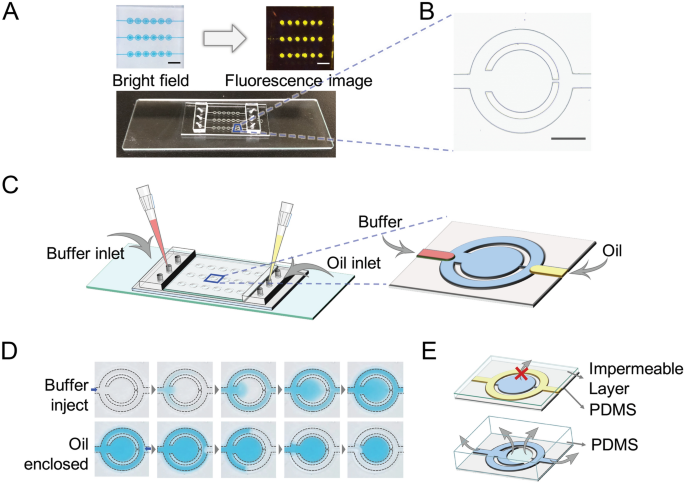This detailed technical illustration is designed to describe the buffering process in a scientific setup. The diagram is divided into five labeled sections, A through E, each illustrating a different aspect of the process.

In section A, entitled "Bright Field Fluorescent Image," there is a square diagram featuring blue dots and an arrow that leads to a black box with yellow dots labeled "Fluorescent Image," accompanied by a relevant photograph.

Section B highlights a circular component that resembles a retina but isn't specified as such.

Section C zooms in on specific instrumentation, showcasing buffer and oil inlets. It features text pointing to the buffer inlet in a red slot and the oil inlet in a yellow slot, both connecting to the circular component shown in section B.

Section D illustrates various states of the circular component as it fills with liquids. Text labels indicate "Buffer Inject" and "Oil Enclosed," showing different levels of liquid from empty to partially full.

Section E highlights the structural composition of the circular component. It includes annotations such as "Impermeable Layer" and "PDMS," with arrows pointing to various layers within the component's cross-section.

This image is predominantly drawn using clear, black outlines, blue and yellow colors for the main components, and red and yellow to highlight specific details, ensuring that the steps and actions are clearly depicted. The overall setup shows how buffer and oil are managed to ensure they do not mix unless desired.